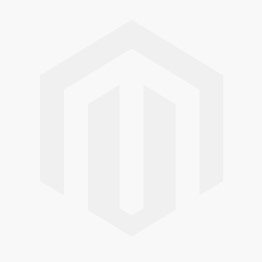This indoor photograph captures a minimalist and stylish room reminiscent of a retail catalog. The room features a light gray wooden-tiled floor and white-painted brick walls, adding a modern yet cozy ambiance. The central focus is a sleek, beige three-seat couch with dark black legs and armrests on both sides, adorned with light gray and white cushions. Hanging prominently on the wall above the couch is a bright pink neon sign shaped like a treble clef, lending a vibrant musical touch to the setting. Flanking the couch are two light-colored wooden bookshelves. The bookshelf on the right holds a soccer ball and various books and trinkets, while the one on the left features a hat hanging off one corner and the edge of a clock peeking into view. To the right of the couch, there is a light-colored wooden desk, providing a subtle yet practical addition to this elegantly simple space.